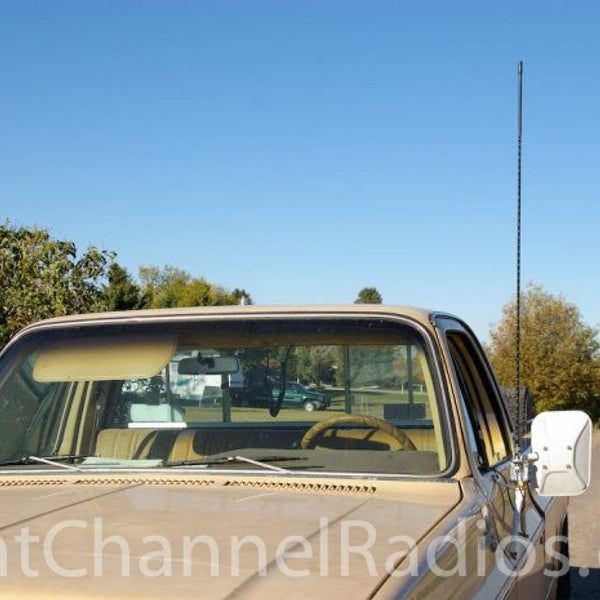This photograph prominently features an old beige pickup truck, viewed from an angle above its hood, emphasizing its windshield and interior. The truck's distinct features include a white side mirror on the left, equipped with an exceptionally tall black antenna projecting upright. The interior showcases a bench seat and steering wheel, both in a matching light brown or beige color. Overlaid at the bottom of the image is a watermark in white text, partially reading "T-Channel Radios."

The truck is parked on what appears to be a dirt road, and the background reveals a mix of a green field, additional parked vehicles—including one towing a trailer or RV—a white building, lush green trees, and a clear blue sky. The setting suggests a casual or camping environment.